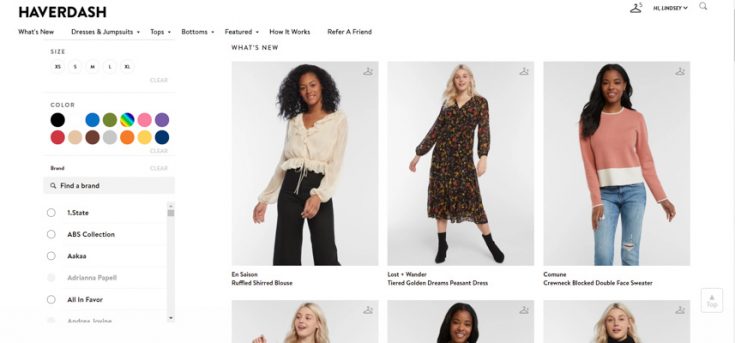This screenshot captures the homepage of the fashion website Havardash. At the top left corner, the site name "HAVARDASH" is prominently displayed in bold, all-capital black font. Directly beneath it, a left-aligned horizontal navigation menu features the following categories: "What's New," "Dresses," "Tops," "Bottoms," "Featured," "How It Works," and "Refer a Friend." 

On the left side of the page, a vertical sidebar menu allows users to filter their search. It starts with the "Size" section, offering five selectable size options arranged horizontally. Following that, the "Color" section displays two rows, each containing seven color swatches for selection. Below the color options, there is a search bar for finding specific brands.

The main content area to the right highlights the "What's New" section, featuring three visible items, with an additional three items partially cut off at the bottom of the screenshot.